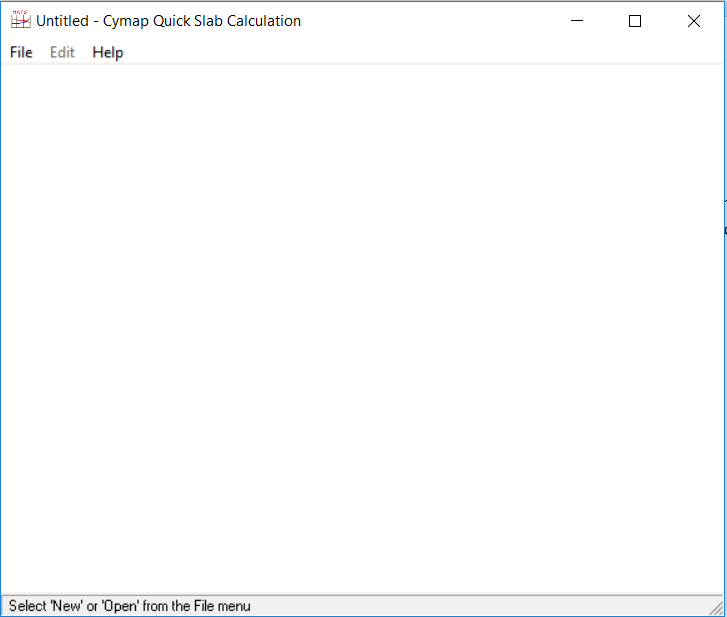The image appears to show a Windows computer application that resembles a text-editing program, possibly Notepad, although its specific functionality suggests it may have different utilities. The application window is labeled "Untitled - CYMAP Quick Slab Calculations." In the top right corner of the window, there are Minimize, Maximize/Restore, and Close buttons.

Directly below the title bar, there is a menu containing "File," "Edit" (grayed out and currently unavailable), and "Help" options. The central portion of the window is entirely blank, indicating that no document is currently open or created.

At the bottom of the interface, instructional text reads: "Select New or Open from the File menu," implying that the user must either start a new document or open an existing one to begin any work within the application. The overall design and components suggest this program is specifically tailored for slab calculations, potentially within the context of civil engineering or architecture.

To summarize, this image showcases a specialized Windows application, "Untitled - CYMAP Quick Slab Calculations," in its initial state, prompting the user to select either 'New' or 'Open' from the File menu to proceed.